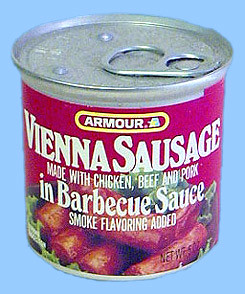This image features a close-up of an Armour brand aluminum can of Vienna Sausage. The can is centrally positioned against a sky blue background, drawing immediate attention. The label is predominantly magenta with bold, white font, displaying the text "Vienna Sausage" prominently. The can indicates that the sausages are made with chicken, beef, and pork, and are immersed in a barbecue sauce with added smoke flavoring. Below the text, there is a vivid image of the sausages nestled on a bed of green lettuce. The Armour brand name sits inside a yellow circle at the top of the label. The can itself has a silver top with a right-facing pull tab and a white edge below the rim.